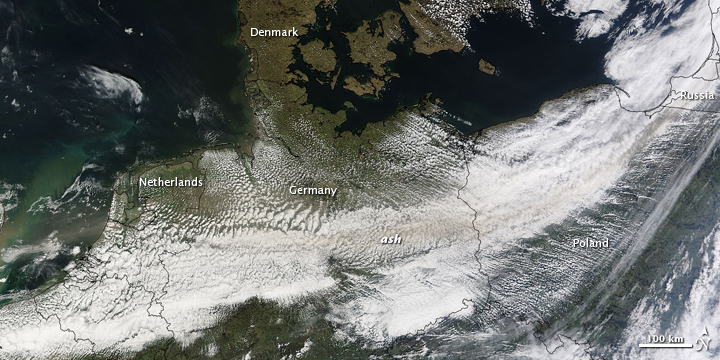This image is a detailed satellite view of parts of Europe, prominently highlighting the countries labeled in white font: the Netherlands on the left, Denmark at the top left, Germany slightly left of center, Poland to the right, and Russia in the upper right corner. The map also features a special designation labeled "ash," indicating a band of grayish-white stretching from the bottom left to the top right of the image, likely representing volcanic ash. This band obscures parts of the landmasses, which include a mix of greenish-brown terrain and greenish-blue water. Faint lines outlining the countries are visible, providing additional geographic context. A scale at the bottom right indicates a distance of 100 kilometers with an arrow pointing north, adding to the map's informative detail.